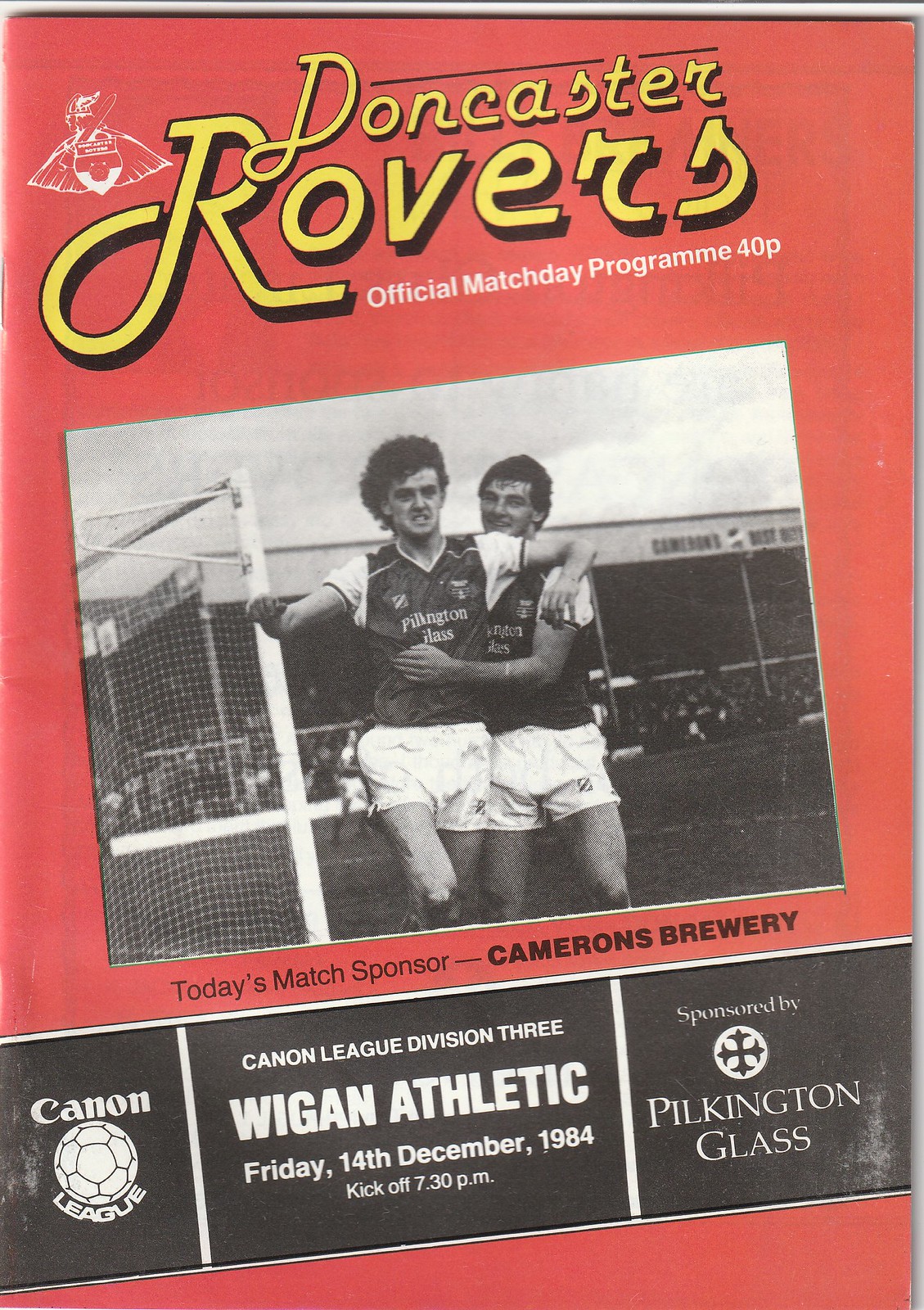The image is of a vintage Doncaster Rovers official match day program, predominantly featuring a striking red background. At the top, in bold, angled yellow letters with black shadows and a retro font, it reads "Doncaster Rovers." To the left of this text, there's an illustration of a Viking with a sword, shield, and cape in white. Beneath the title, in smaller white letters, it states "Official Match Day Program 40P."

Central to the program cover is a black and white image depicting two soccer players, who appear to be wearing white shorts and possibly black and white tops. These players are positioned towards the front, with the stadium, including the crowd, goalposts, and soccer pitch, visible in the background. One player is hugging the other, and both are looking directly towards the viewer. Below this central image, in black letters, it reads "Today's Match Sponsor Cameron's Brewery."

At the bottom of the brochure, a black bar runs across with various advertisements and match details. On the left side of the bar, it says "Cannon" with an image of a soccer ball and "League" beneath it. Central to the bar, the text reads "Cannon League Division III Wigan Athletic, Friday 14th December 1984, kickoff 7.30 p.m." On the right side, it says "Sponsored by Pilkington Glass" with a circular logo featuring a black cross.